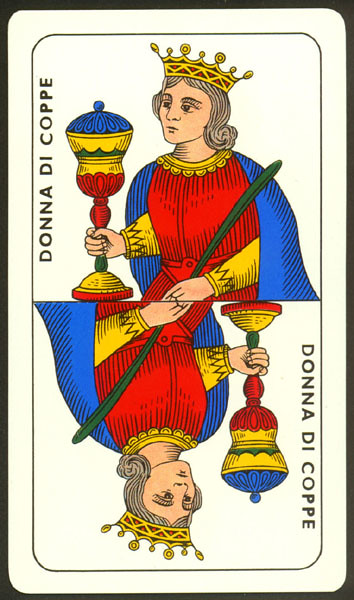The image features a portrait-oriented card framed in black. At the center is a detailed depiction of what appears to be the Queen of Cups. She is characterized by her long, gray, curled hair and adorned with a symbolic gold crown. Her attire is richly detailed, featuring a red vestment and a blue cape, with intricate gold lace around her throat. Beneath the vestment, a golden shirt is partially visible. 

In her right hand, the Queen holds a large, ceremonial chalice, intricately decorated with patterns in gold, red, green, and blue colors. In her left hand, she appears to be holding a green leaf-like object. The chalice’s design is elaborate and eye-catching, suggesting it has significant symbolic value.

On the left side of the card, the text "Donna Di Coppe" is inscribed, a name that also appears in an inverted orientation at the bottom, maintaining symmetry. The Queen gazes thoughtfully at the name "Donna Di Coppe" while also appearing to focus intently on the detailed chalice in her right hand.